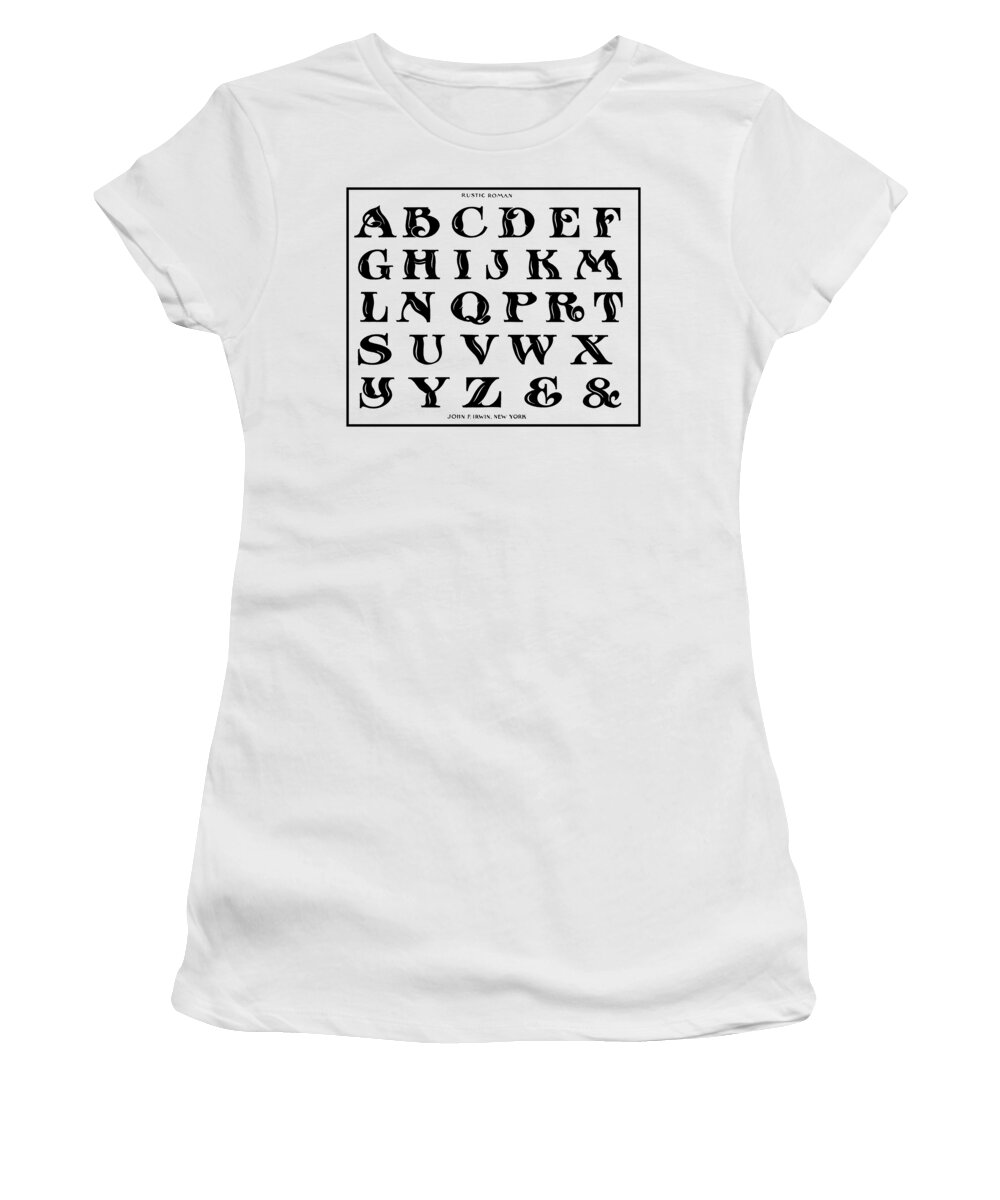This is a photograph of a short-sleeved white t-shirt designed for women, identifiable by its sleeves ending right at the armpit. The t-shirt features a crew neck and is made from white fabric. In the middle of the shirt, there is a prominent black square box containing a distinctive black and white graphic of the alphabet. The letters are arranged over five rows, with each row featuring six hand-drawn style letters. The first row displays A, B, C, D, E, F, while the last row ends with Y, Z followed by two ampersand (&) symbols. Below the alphabet graphic, the text "New York" is partially visible, although the first part of the phrase is unclear. The overall aesthetic is casual with a playful, almost wavy font style for the alphabet, and the image background is solid white, resembling a typical product image you'd find on a shopping website.